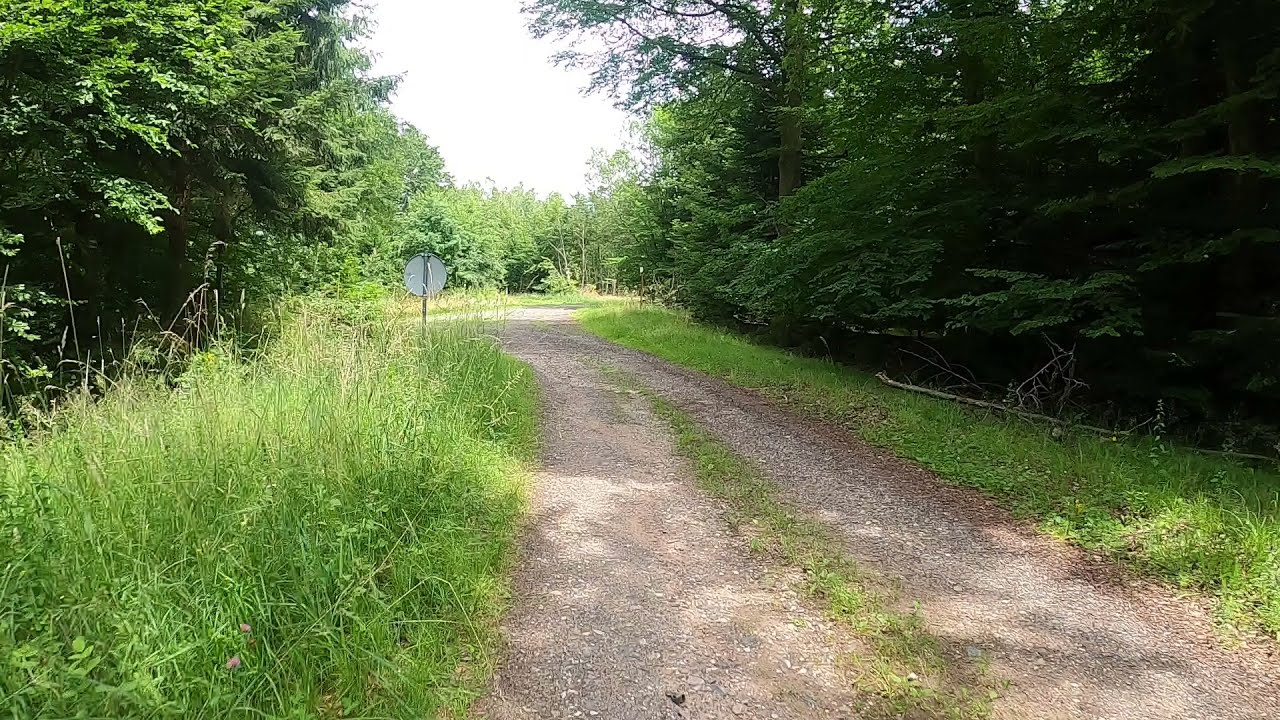This photograph captures a meandering gravel pathway that cuts through an area of tall, wild grass and lush green forest. The pathway, brown in color and interspersed with pebbles and patches of grass, curves towards the right further ahead. The left and right sides of the pathway are lined with tall, vibrant green grass that transitions into dense trees in the background. These trees cast intricate shadows onto the pathway and surrounding grass, highlighted by beams of sunlight. A silver signboard is visible on the left side near an intersection. The sky overhead is a bright white, suggesting it is either morning or noon, and the overall scene is bathed in clear, natural light.